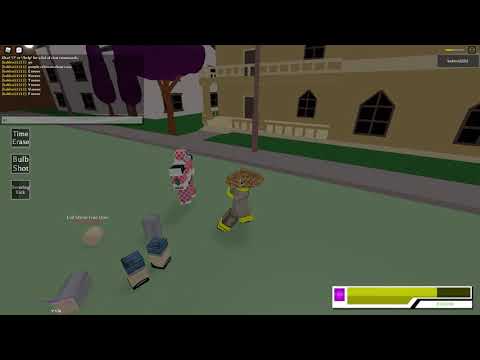This image is a screen capture of a primitive, blocky video game with a black header and footer. The game world features a simplistic, three-dimensional landscape. In the foreground, there are two blocky characters standing on a mint-green courtyard. The character on the right is gray with yellow accents and has a brown, triangular element on the top of its head, possibly a hat. The character on the left is pink with black polka dots and has some white blocks on it. In the lower left of the screen, various geometric shapes like a white ball, gray cylinders, and blue and white rectangles, some of which appear to be knocked over, suggest interactive game elements. The background showcases a yellowish-tan building with blocky windows and a railing in front, hinting at a possible two-story structure. Behind this building, there are additional trees with purple leaves obscuring a white two-story building. In the upper left corner, there's a chat or display possibly revealing ongoing game details, although it's not entirely legible. A progress bar with purple, yellow, and black segments is located in the lower right. Icons labeled "bulb," "shoot," and "time" indicate potential in-game actions or tools.